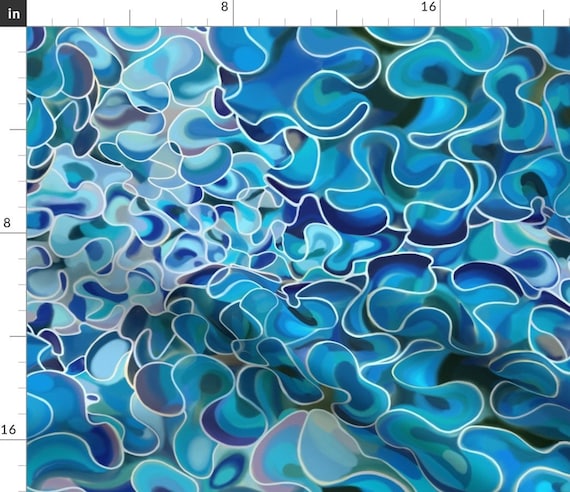This abstract graphic features dynamic swirls and curves reminiscent of ribbon, bordered by squiggly white lines that delineate various sections. The vibrant composition prominently showcases multiple shades of blue, ranging from royal blue to turquoise, interspersed with light blue and hints of dark blue. Accents of mauve, pink, and a small amount of green at the bottom add depth to the visual. Notably, the image bears a striking resemblance to refracted light patterns seen at the bottom of a pool, but with smoother, less angular lines. Along the top and left sides are measurement marks, extending to 8 and 16 inches, suggesting a deliberate layout. A small square in the top left corner contains white text, indicating precise dimensions and reinforcing the structured aspect of this visually fluid and colorful creation.